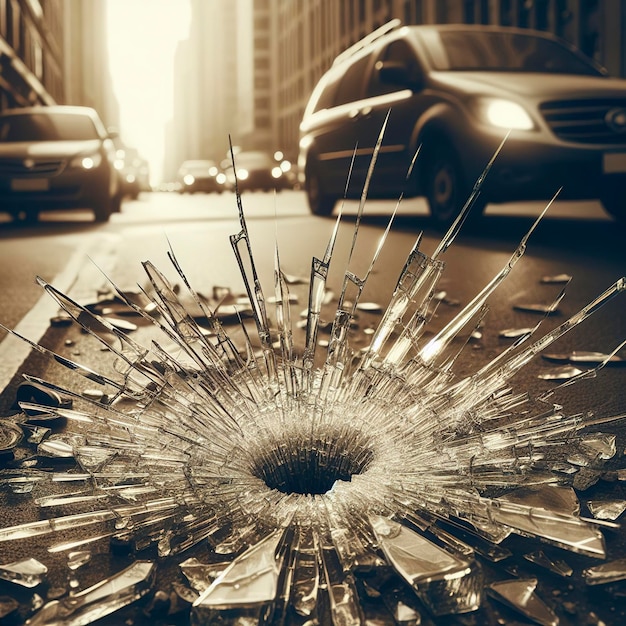This is a digitally altered, stylized photo captured from a low vantage point on a busy roadway. The image, viewed through an amber filter, features a surreal scene where the middle of the road displays a large pit surrounded by shattered glass shards spiking out like needles, creating a dramatic visual effect. The amber-hued environment adds to the surrealism, contrasting sharply with the crystal-clear glass fragments. Vehicles, including an SUV in the foreground, approach the viewer with their headlights on, suggesting the time is near sunset. The street is flanked by tall buildings filled with numerous windows, lining both sides and receding into the distance. The white lines on the road are clearly visible, and the far distance is shrouded in what appears to be smog or smoke, adding another layer of depth to this otherworldly landscape.